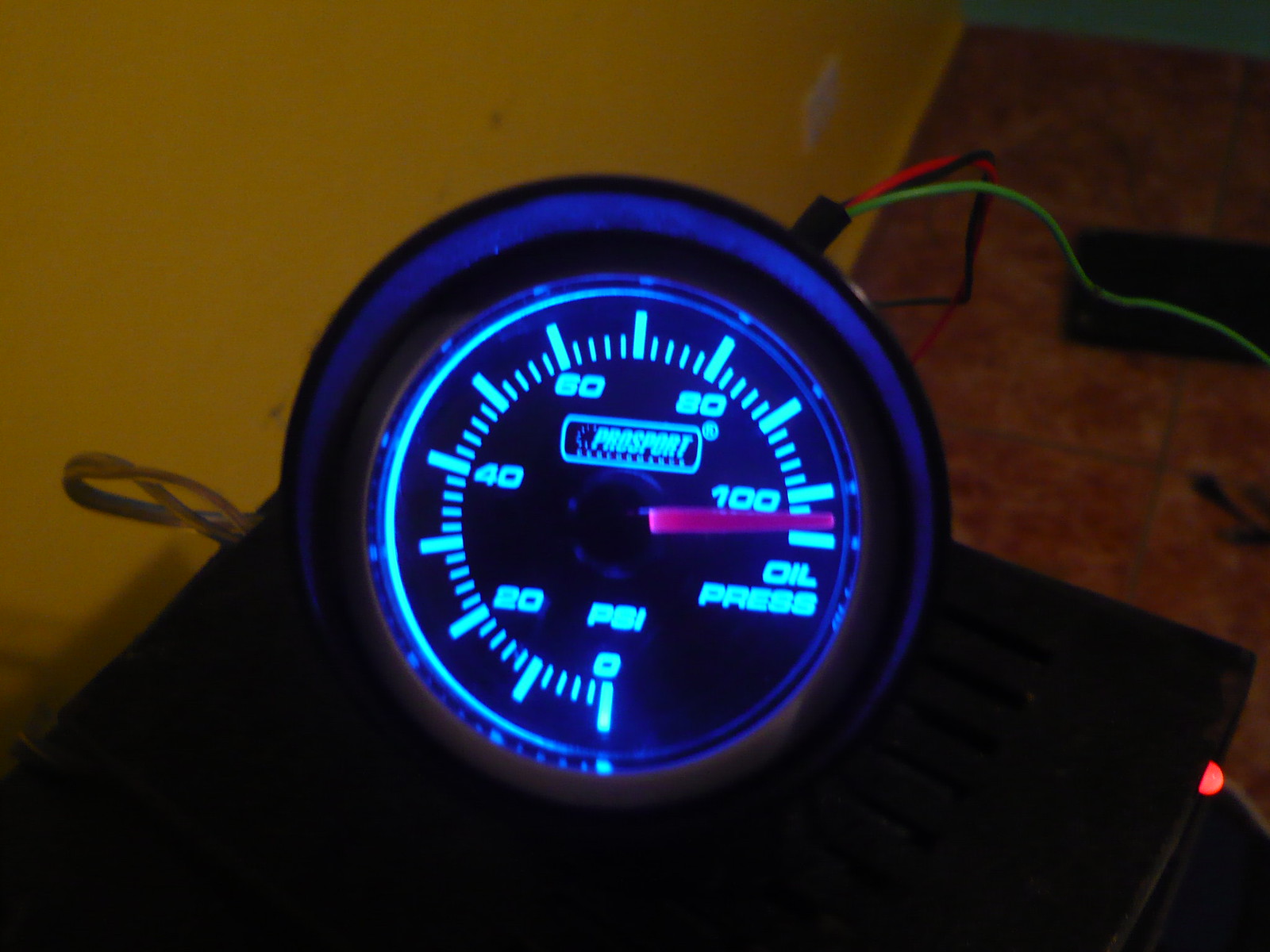The image captures a PSI meter of an oil press, enveloped in a dimly lit environment which makes discerning details a challenge. The meter itself is distinctly illuminated by neon lights, highlighting both the numerical markers and the meter's border. Two cords, one orange and one green, are visible on the side of the meter. The PSI meter features a prominent red arrow indicating the current pressure reading, past the 100 PSI mark. The display reads from 0 to over 100 PSI, with the maximum label marked "oil press." The brand name, "Crossport," is partially visible at the top center, though the remaining text is too blurry to decipher. The glowing blue light adds a striking contrast to the otherwise dark setting. On the left, an additional cord with a loop is noticeable. The backdrop appears to be a yellowish-green wall, but the true color remains indistinct due to the low lighting.